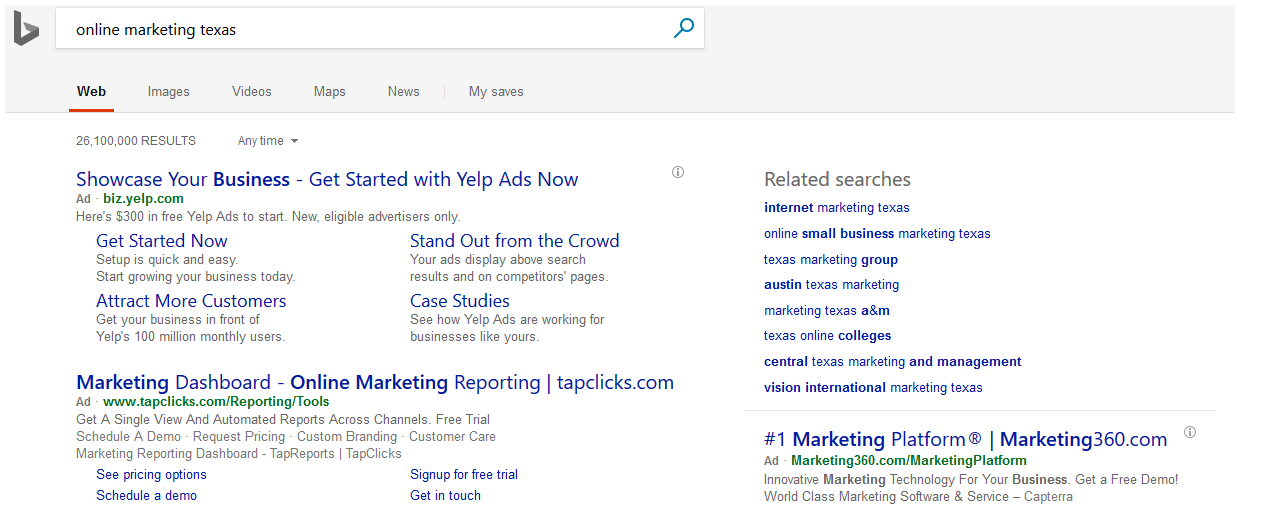The image is a screenshot from a website displayed against a white backdrop. At the top, there's a roughly one-inch thick gray-white bar spanning across the page. In the upper left corner, a stylized lowercase 'b' in black is constructed from straight lines. To its right is a white search bar with the text "Online Marketing Texas" in black. This search bar extends halfway across the page and ends with a blue magnifying glass icon on its right.

Below this bar, a menu appears with black text: "Web," "Images," "Videos," "Maps," "News," and "My Saves." The word "Web" is bolded and underlined in red. In the white section beneath, the number "26,100,000 results" is displayed in black on the left side. To the right, "Anytime" is shown with a drop-down icon next to it.

Further down, there's an advertisement from Yelp. The headline in blue reads, "Showcase your business—get started with Yelp ads now," followed by the word "Ad" in black. The URL "biz.yelp.com" appears in green. The ad elaborates in black text, offering "$300 in free Yelp ads to start. New, eligible advertisers only." Below, a blue link says, "Get started now," accompanied by "Setup is quick and easy." The text continues, "Start growing your business today," and a blue link reading, "Attract more customers" follows. Further details in black state, "Get your business in front of Yelp's 100 million monthly users," located to the right of another blue link, "Stand out from the crowd." Additional black text notes, "Your ads display above search results and on competitors' pages," with another blue link, "Case studies," suggesting, "See how Yelp ads are working for businesses like yours."

Further down, another blue link reads, "Marketing dashboard - online marketing and reporting," followed by "TapClicks.com" in black. The ad section mentions, "www.tapclicks.com" in green, listing features like "Get a single view and automated report across channels. Free trial. Schedule a demo. Request pricing. Custom branding. Customer care. Marketing reporting dashboard. And top reports." 

A blue link prompts users to "See pricing options," and to its right, another link says, "Sign up for free trial." Below, the text urges, "Schedule a demo" on the left, with "Get in touch" in blue on the right.

On the right side, under the "Related searches" header in black, several blue links are listed: "Internet Marketing Texas," "Online Small Businesses Marketing Texas," "Texas Marketing Group," "Austin Texas Marketing," "Marketing Texas A&M," "Texas Online Colleges," "Central Texas Marketing and Management," and "Vision International Marketing Texas." Another blue link states, "#1 Marketing Platform," beside a reserved rights symbol, and the URL "Marketing360.com" in black text. Below, "Marketing360.com/Marketing Platform" appears in green. The ad description reads, "Innovative Marketing Technology for Your Business. Get a free demo!" followed by "World Class Marketing Software and Service" and possibly "CAPTEUR" in black.